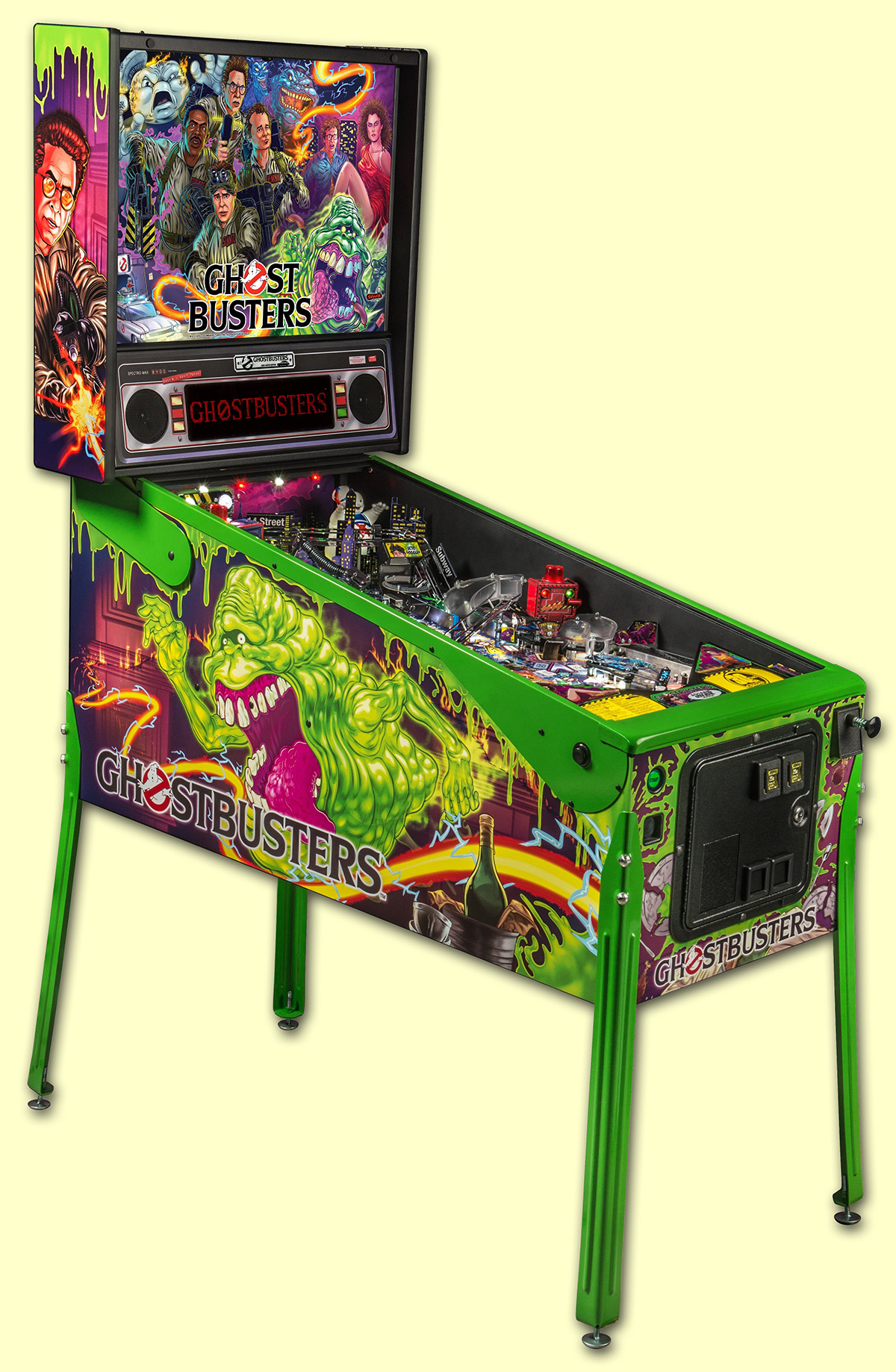The image features a vintage Ghostbusters-themed pinball machine prominently positioned diagonally from the top left to the bottom right of the frame. The machine, primarily green in color, stands on four green legs and showcases vibrant graphics in purple and yellow. The word "Ghostbusters" is written in grey on the top panel, the side, and the front of the machine. A distinctive green, blob-like monster with white teeth and a pink tongue, reminiscent of characters from the Ghostbusters franchise, is illustrated on the side. There are also depictions of characters from the movie at the top of the machine. The top section features a glass-covered scoreboard, and there is a red sign visible as well. The coin insertion area has a black panel, and green lights adorn the bottom of the machine. The entire setup is placed against a light beige or yellow background, giving it a classic arcade gaming environment.